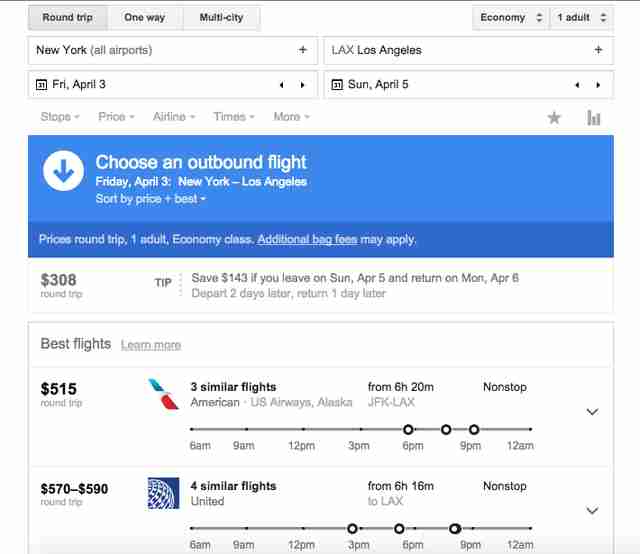A travel itinerary search form set against a white background shows a round-trip selection checked, with options for one-way and multi-city travel left unchecked. The traveler is booking an economy class ticket for one adult, departing from New York on Friday, April 3rd, to Los Angeles, and returning on Sunday, April 5th.

A blue-highlighted box urges the user to "choose an outbound flight" for Friday, April 3rd, from New York to LA, sorted by "price and best." The search results indicate that round-trip economy fares for one adult begin at $308, with extra baggage fees potentially applicable.

A tip suggests saving $143 by adjusting travel dates to depart on Sunday, April 5th, and return on Monday, April 6th, moving the departure two days later and the return one day later. Other flight options include three similar flights priced at $515 each, offered by U.S. Airways, Alaska, and American Airlines. Additional options range from $570 to $590 for round trips, with four similar, nonstop flights available. The detailed pricing and flight options information ends at this point.